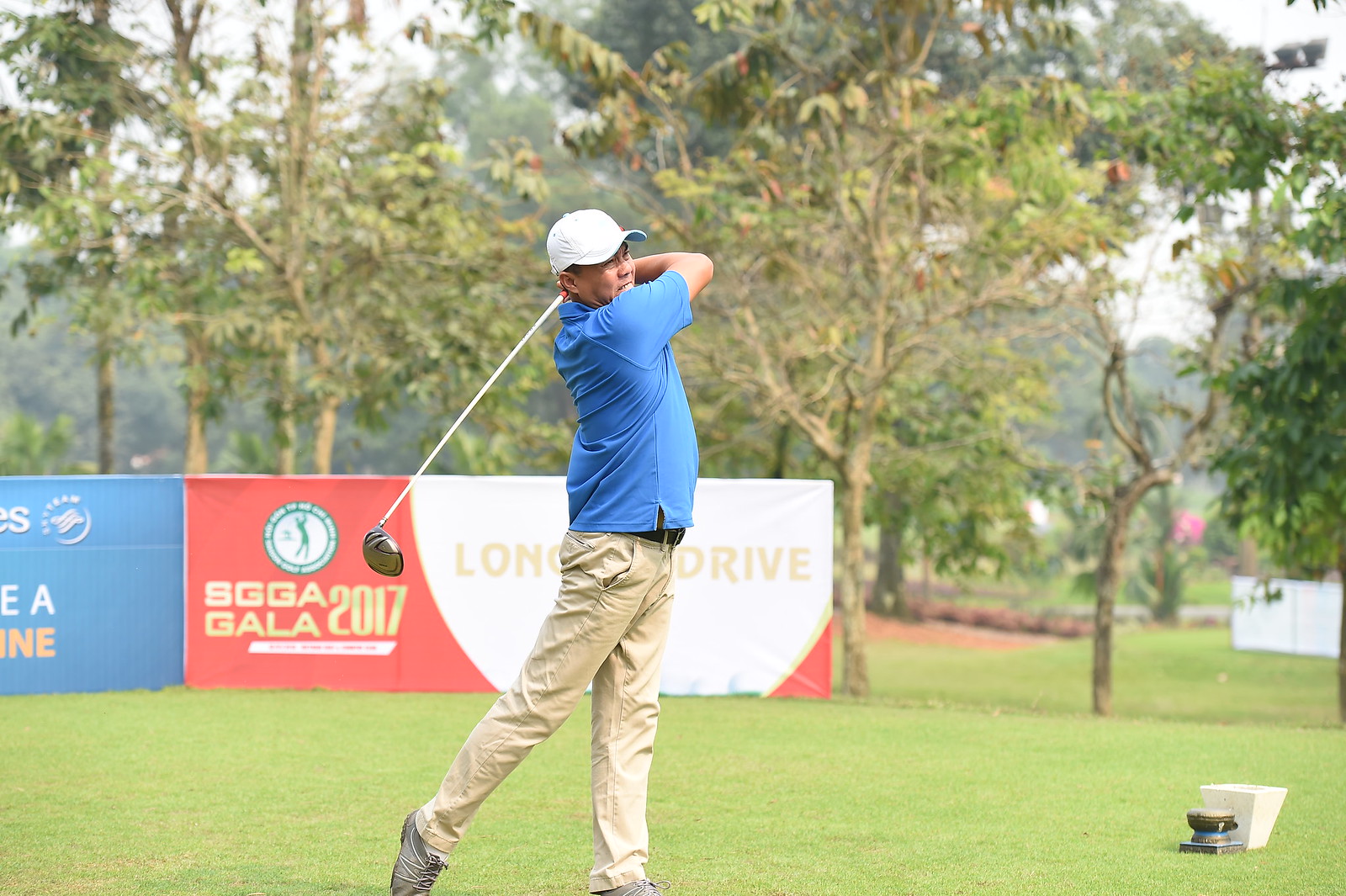This image depicts an Asian man in mid-swing on a lush, well-maintained golf course. He is dressed in a white baseball cap, a blue polo shirt, light khaki pants, and gray athletic shoes. With a focused gaze, he follows the trajectory of his recently struck golf ball, his club still elevated behind his back, capturing the moment of his powerful swing. The vibrant green grass beneath him contrasts beautifully with the surrounding dense trees, indicating a serene and clear day. Behind the golfer, sponsor banners can be seen, including a prominent red and white one bearing the gold inscription "SGGA Gala 2017." Additionally, the words "Long Drive" hint at a specific competition or event category. In the foreground, there appear to be two indistinct objects that resemble vases. The overall setting suggests a professionally organized golf event, underscored by the immaculate condition of the course and the visible sponsorship signage.